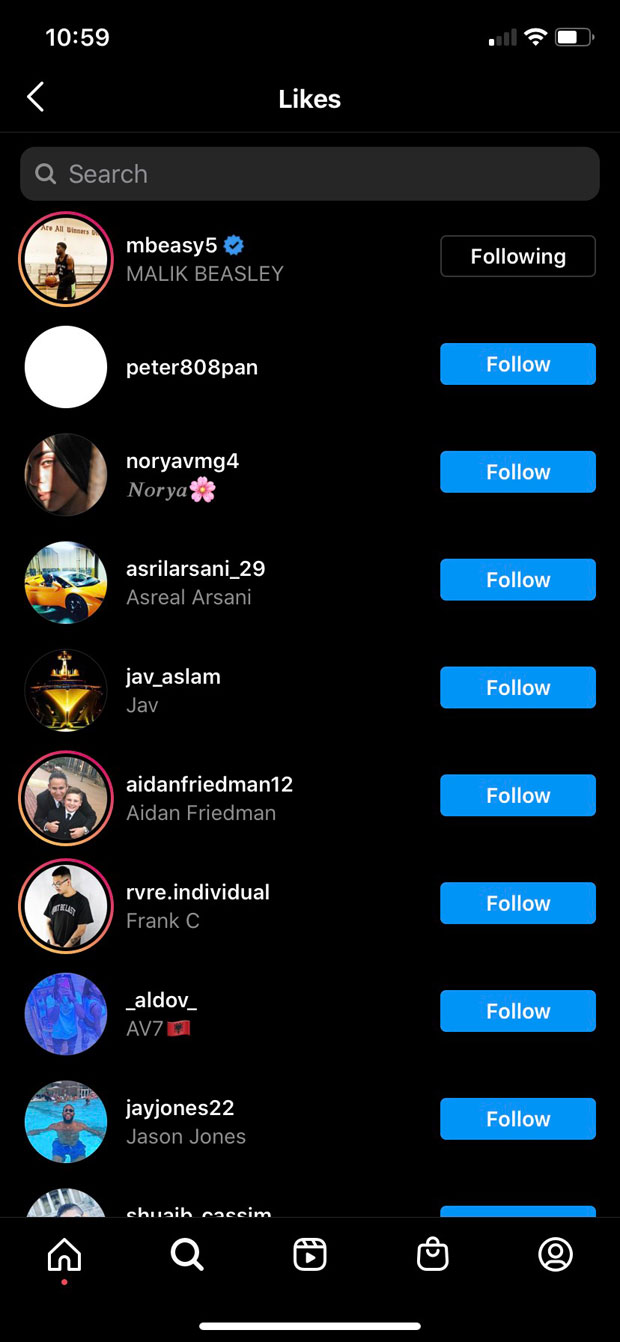The image displays a roster of names against a black background. At the very top left corner, the time is shown as 10:59. To the right on the same line, there are signal and battery notifications in white. Below this, centrally positioned, is the word "Likes". Just underneath "Likes", a search bar with an hourglass icon on the left is visible. 

Beneath the search bar, there are pictures of various people and logos, each accompanied by a name. At the top of the list is Malik Beasy, with a white "Following" label adjacent to the name. Following Malik Beasy, the names listed downward are: Peter808PAN, NoriAVMG4 with a pink flower petal icon next to "Noria", S.Rillasani29, Arsani, Jav Aslam with the nickname "Jav", Aiden Friedman 12 with the complete name as "Aiden Friedman", RVRE.Individual, Frank C. Aldove AV7 with a red icon, and Jade Jones 22 with the name "Jason Jones". Each of these names has a blue button labeled "Follow" in white lettering to its right.